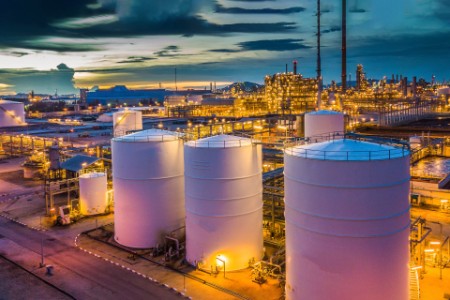The photograph depicts an industrial plant, possibly a water treatment or petroleum distribution facility, captured just after sunset. The sky features a mix of blues, grays, and some lingering orange hues, giving it a slightly foreboding yet picturesque appearance. The entire area is illuminated with yellow lights across the structures and streets, providing a warm glow against the twilight backdrop.

Central to the image are three large, white cylindrical tanks prominently positioned from right to left in the foreground. A road runs diagonally from the bottom left corner, passing by these tanks. In the background, there are additional smaller white tanks, arranged in a staggered fashion. The facility is replete with a network of piping and fencing, enhancing its industrial complexity.

A hint of water is noticeable on the right-hand side of the photo, reflected by the lights, adding another layer of texture to the scene. In the far distance, a mountain range outlines the horizon, completing the composition. The overall atmosphere suggests a bustling, well-lit industrial hub set against the transitioning colors of the evening sky.